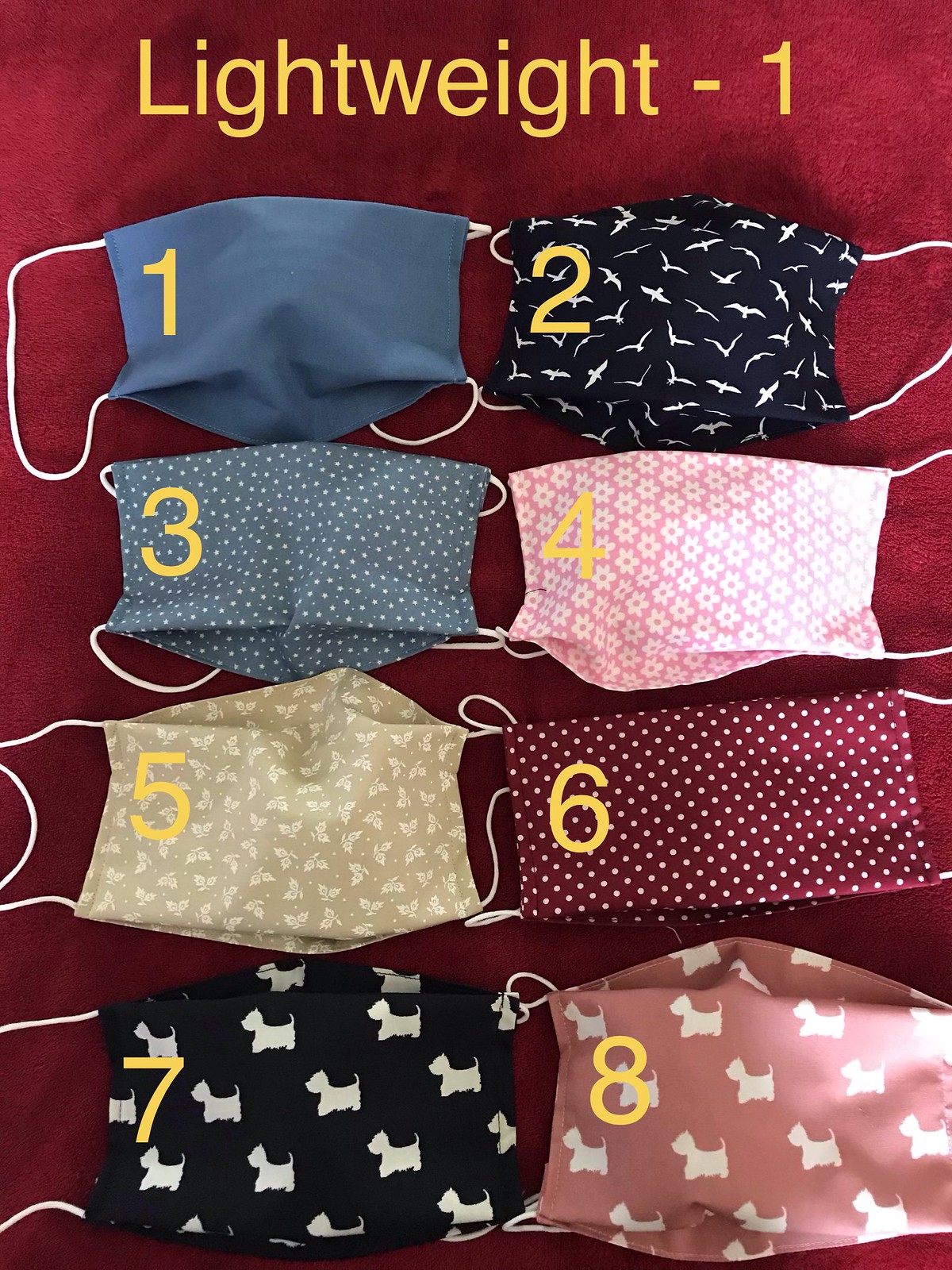The image displays eight distinct fabric masks arranged on a red carpet-like background, each labeled in yellow text. At the top, white text reads "Lightweight-1." The masks are organized in four rows, with two masks per row. The numbers are positioned as follows: 1, 3, 5, 7 on the left and 2, 4, 6, 8 on the right.

Each mask has a unique design:
1. A solid blue mask.
2. A black mask with white birds.
3. A blue mask with white polka dots.
4. A pink mask featuring white flowers.
5. A green mask adorned with butterflies and leaves.
6. A red mask with white circles.
7. A black mask decorated with white terrier-like dogs.
8. A pink mask with the same white terrier-like dogs as mask 7.

Each mask has white strings on the sides, suggesting they are handmade fabric masks similar to those worn during the COVID-19 pandemic.